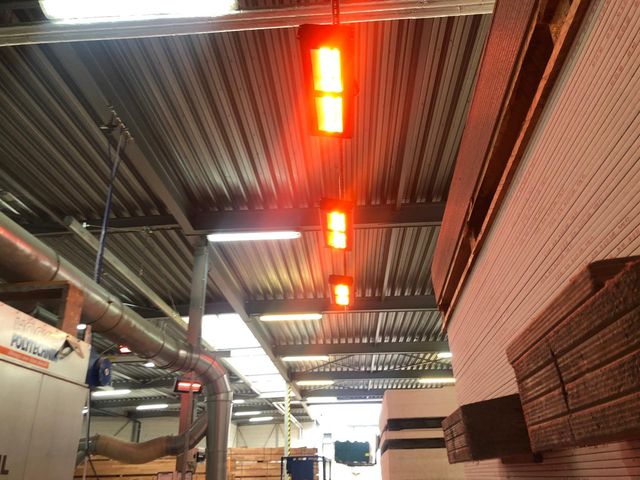The photograph showcases the interior of a large, industrial warehouse. The focal point is the ceiling, which is constructed of clean, corrugated steel with distinct, parallel lines. The ceiling also features several ductworks, primarily on the left, running horizontally and vertically. Hanging from the ceiling is a long, reddish-yellow light emitting a warm glow.

The walls of the warehouse are predominantly white with isolated patches of exposed bricks, enhancing the industrial aesthetic. On the right side of the image, there are numerous stacked wooden pallets and beige materials, possibly shelves or boxes. A large steel pipe and an adjacent machine can also be seen on the left side of the image.

Additional lighting is provided by fluorescent lights scattered throughout the warehouse. The ceiling may have either an open section or several flat windows. The overall impression is that of a spacious, busy industrial setting, with various functional elements seamlessly integrated into its infrastructure.